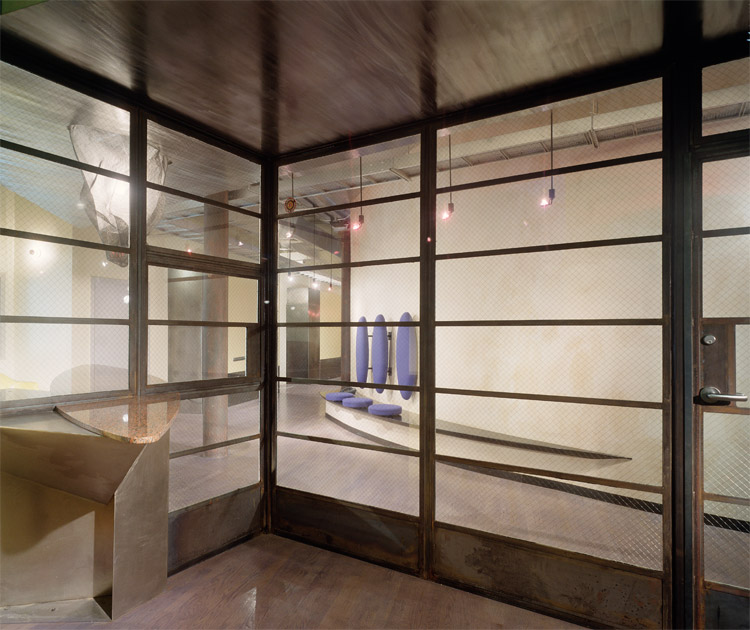This photograph captures the interior of a modern, glass-enclosed room within a building. The room features striking lines and a contemporary design, with metal and glass walls that offer a clear view into adjacent rooms and a connecting hallway. The interiors boast dark wooden floors and ceilings, complemented by off-white walls and stick lighting. The visible hallway outside the enclosure has a glossy, hard gray surface and curved walls that lead out of sight. The left side of the room reveals furniture protruding from the corner, while the right side wall features vertically oriented blue and purple art installations, with small matching discs beneath them. The glass enclosure includes a door on the left, equipped with a visible 30-lock mechanism and wire netting reinforcement. This space, with no people in sight, feels like a blend of an office, library, or art studio, reflecting both functionality and artistic expression.